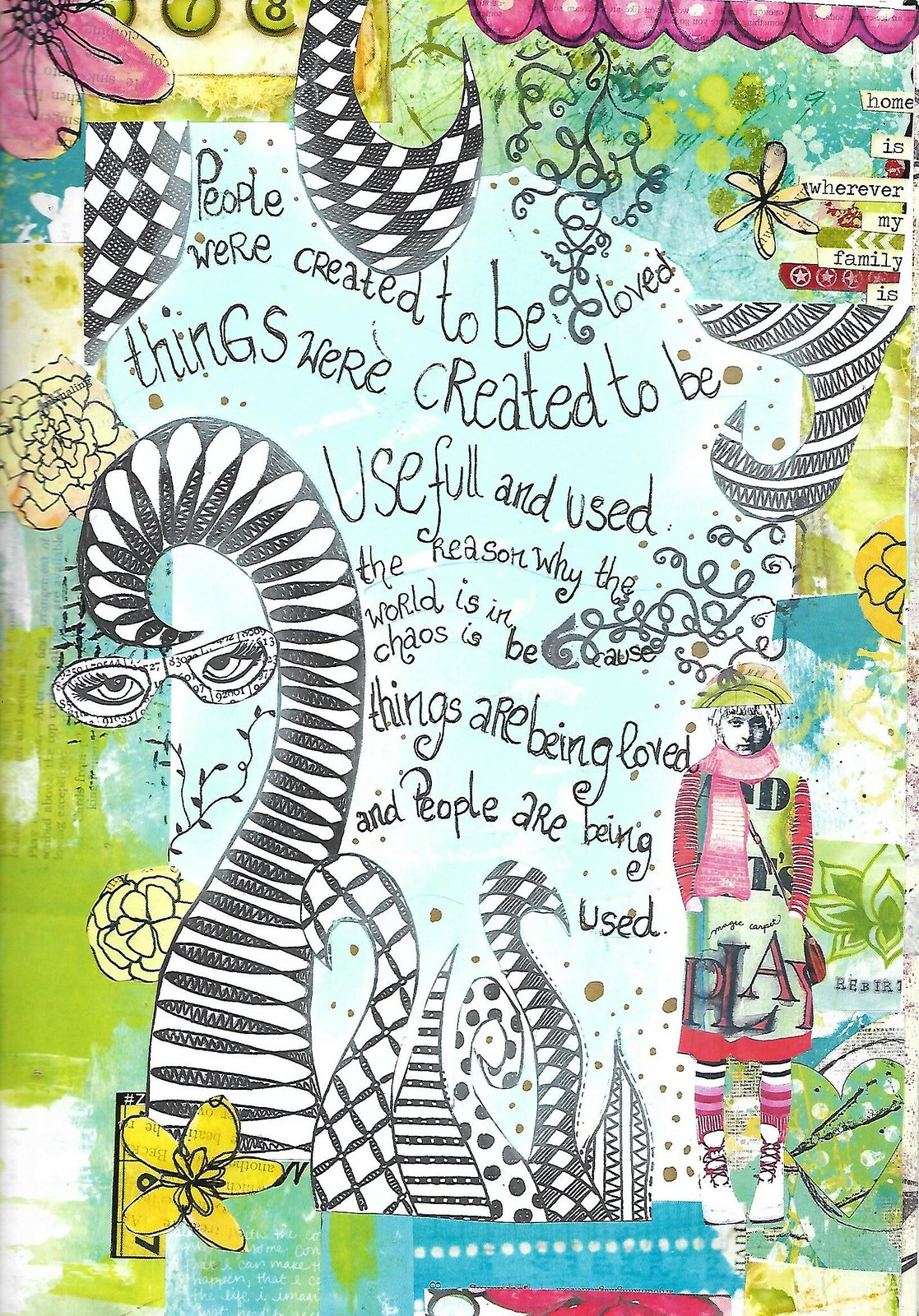This vibrant and intricate piece of artwork features a surreal drawing filled with an array of colors including black and white, various shades of blue, green, yellow, pink, fuchsia, and purple. Central to the image is handwritten black text that reads, "Home is wherever my family is," and, "People were created to be loved, things were created to be useful and used. The reason why the world is in chaos is because things are being loved and people are being used." The artwork includes several distinctive elements: a large snake with human eyes hidden behind sunglasses, flowers that resemble doodles, a woman in a very colorful dress with purple socks, white shoes, and a yellow hat, and a pair of eyeglasses with eyeballs looking through the lenses without an accompanying head or face. The composition of the artwork, paired with these unique details, makes it one of the more bizarre and captivating images you might encounter. The text is centrally placed, making it a focal point amidst the colorful chaos.